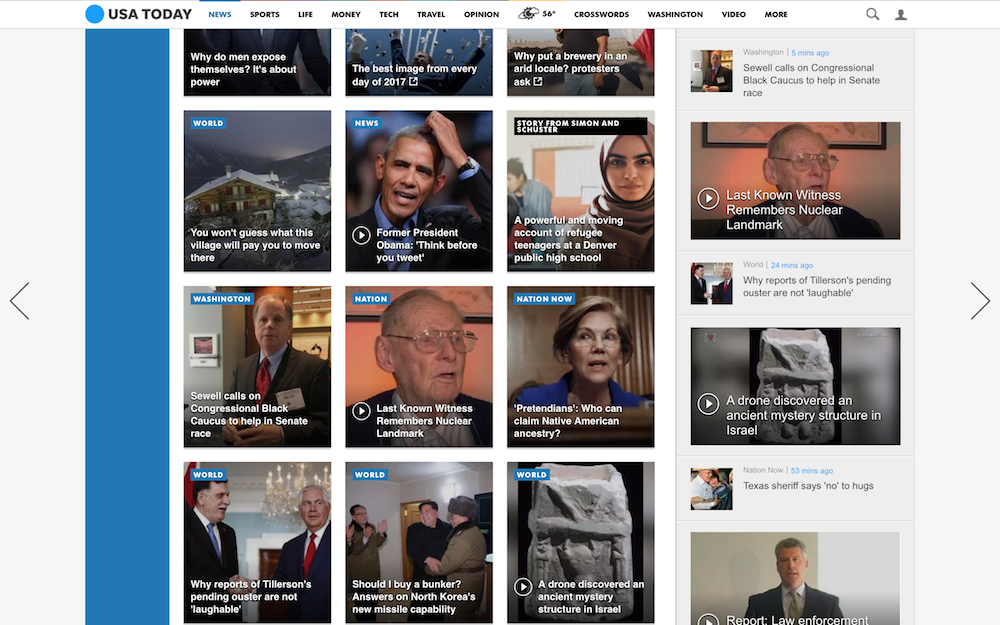The image displays a USA Today webpage, showcasing various article categories including News, Sports, Life, Money, Tech, Travel, Opinion, Crosswords, Washington, Video, and More. Prominently featured are headlines highlighting a range of compelling stories. Key headlines include: "Why do men expose themselves? It's about power," "The best images from every day of 2017," and "Why put a brewery in an arid locale? Protesters ask." Another headline teases a unique story with, "You won't guess what this village will pay you to move there." The page also features an opinion piece from former President Obama titled "Think before you tweet," and a story from Simon & Schuster about refugee teenagers at a Denver public high school, described as "a powerful and moving account." Additional articles cover topics such as Sewell calling on the Congressional Black Caucus to help address racial issues, a last known witness recalling a nuclear landmark, and a discussion on who can claim Native American ancestry.